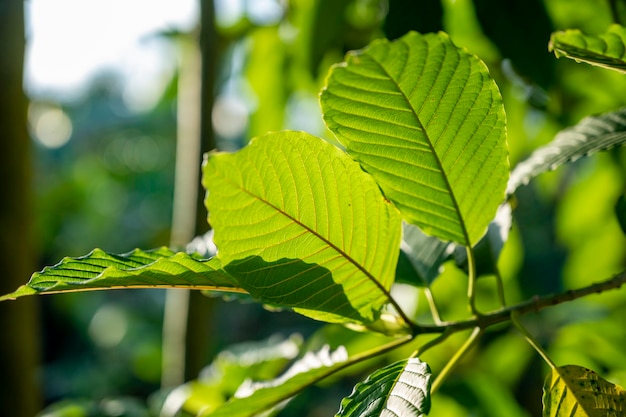In this close-up photograph, a branch of a green plant is captured in intricate detail. The picture highlights the slender, silvery stems and dark brown branches, suggesting they are the newest and youngest parts of the plant. The oblong, healthy-looking leaves exhibit visible veins, adding to their lush appearance, although one leaf near the bottom shows a yellowish hue, potentially from insufficient sunlight. The composition is focused on a group of leaves at the tip of the branch, creating a sense of intimacy and detail. The background is a soft blur, giving the impression of either an indoor or outdoor setting, with a windowsill possibly hinted at in the backdrop. Sunlight is evident, casting delicate shadows of adjacent leaves and adding a natural glow to the greenery. There are subtle hints of thicker branches or tree trunks in the distance, adding depth to the photograph and suggesting a more extensive foliage environment.